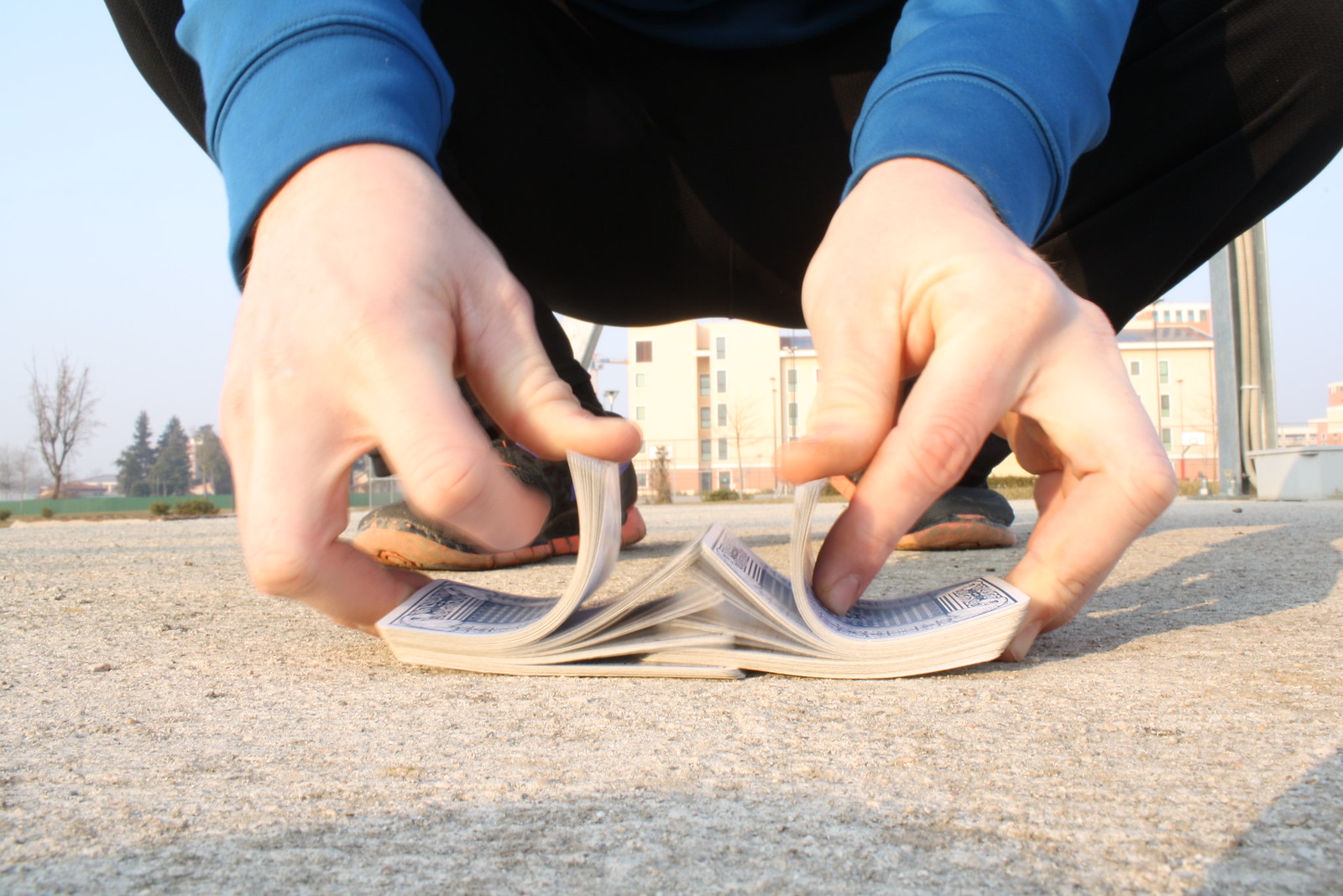In this close-up photograph taken from ground level, we observe a male individual skillfully shuffling a deck of cards on a sandy-colored, irregular concrete surface. The person, identifiable by their fair skin, is clad in a long-sleeved blue sweatshirt, black pants, and black sneakers with orange soles. Only the lower portion of their body and their hands are visible, as they squat with knees pointed outward, splitting the deck into two halves and intermixing the cards. The cards themselves are white, adorned with a blue and white design on the back.

Behind and between their legs stands a multi-level building, likely a hotel, with a distinct architecture. The building features a red brick base, upper floors constructed from yellow brick, and a black vaulted roof. To the right, a patch of green grass houses three tall evergreen trees and a bare-branched deciduous tree. A yellow construction crane is positioned to the left of the building, towering over the scene.